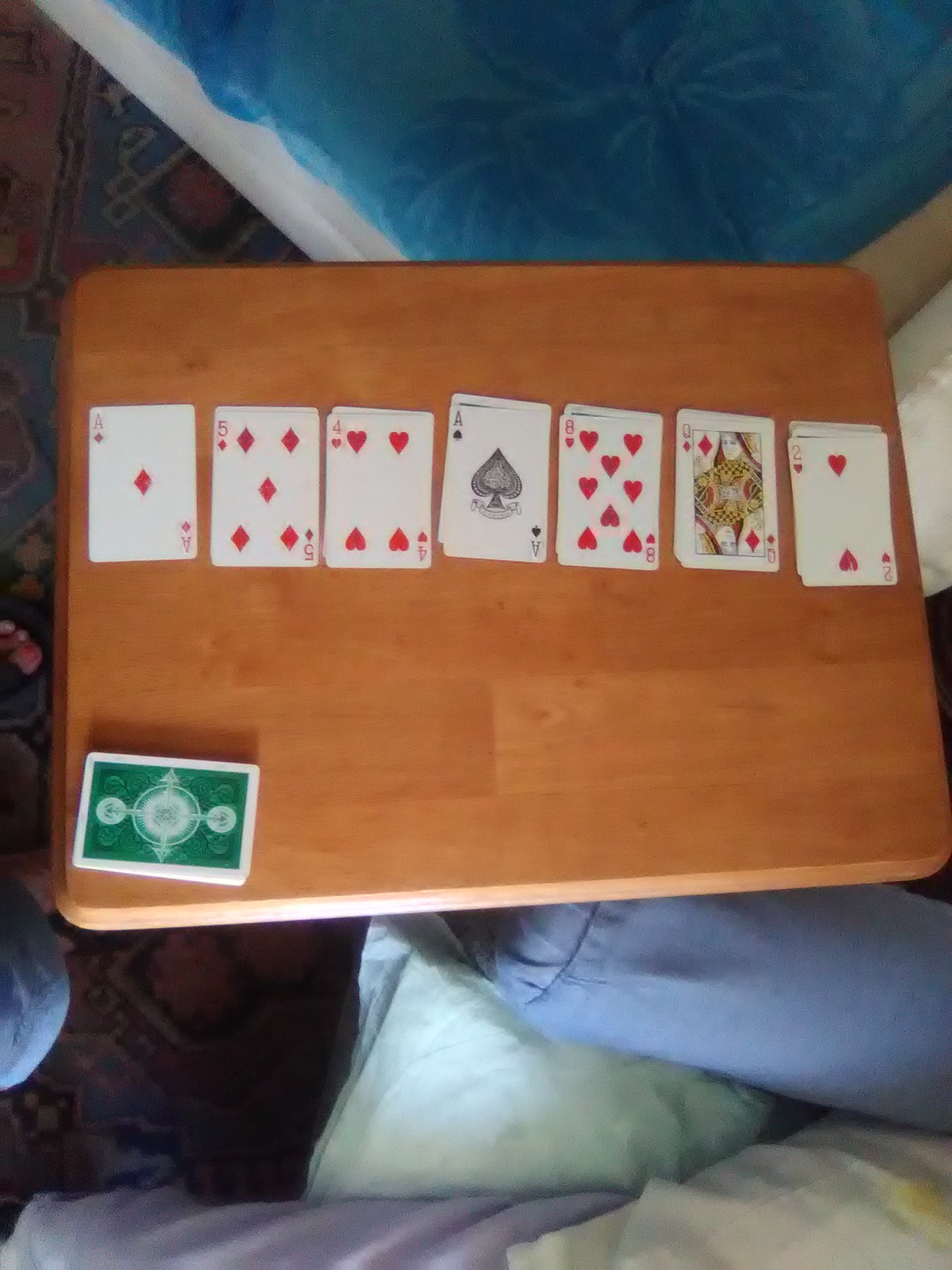The image depicts a light wooden lap desk or a small table placed just above a variety of pillow cushions of different sizes, suggesting a cozy and informal setting. Behind the table, a wall partially covered with a blue fabric or screen is visible, adding a subtle backdrop to the scene.

On the table, seven carefully arranged stacks of playing cards are spread from left to right. The first card, an Ace of Diamonds, is prominently positioned on the left. Next to it, a Five of Diamonds is partly visible with additional cards tucked behind it. Following this sequence, a Four of Hearts appears next to the Five, also having several cards behind it. An Ace of Spades is situated after the Four, accompanied by more hidden cards. Then comes an Eight of Hearts with its own concealed cards. Next to it, a Queen of Diamonds stands out, again with cards behind it. Finally, a Two of Hearts concludes the series on the right side, also backed by more cards.

Below these seven stacks is a deck of cards with an eye-catching cover, featuring green shapes accented with white trim. The detailed arrangement and varied card styles suggest a moment of strategic gameplay or an ongoing solitaire session.